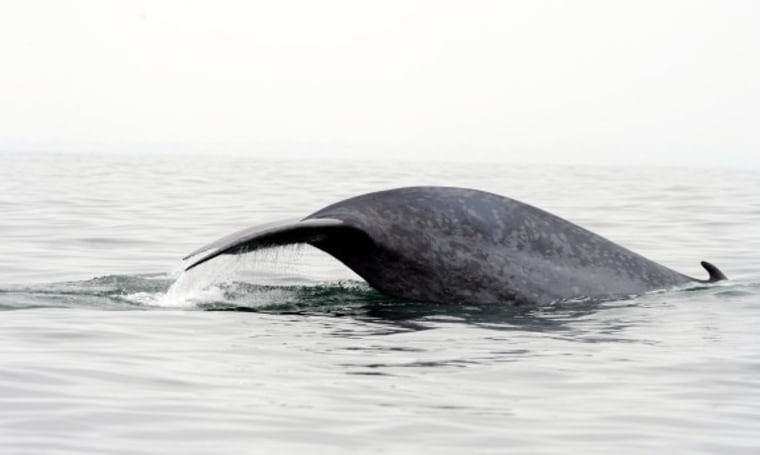This black-and-white photograph captures a serene, overcast scene of a vast, calm ocean with pale gray waves reflecting the sky above. Dominating the center of the image is the tail of a large aquatic animal, likely a whale or a similar creature, as it descends into the water. The creature's skin is a darker gray, contrasting against the muted backdrop. Water drips off the tail, creating small waves and ripples around it. A slight fin is visible near the front, just starting to submerge, while two larger tail fins, or flippers, are prominently displayed, relaxed to either side. The overall atmosphere is tranquil, with the only disturbance being where the majestic animal interacts with the still water.